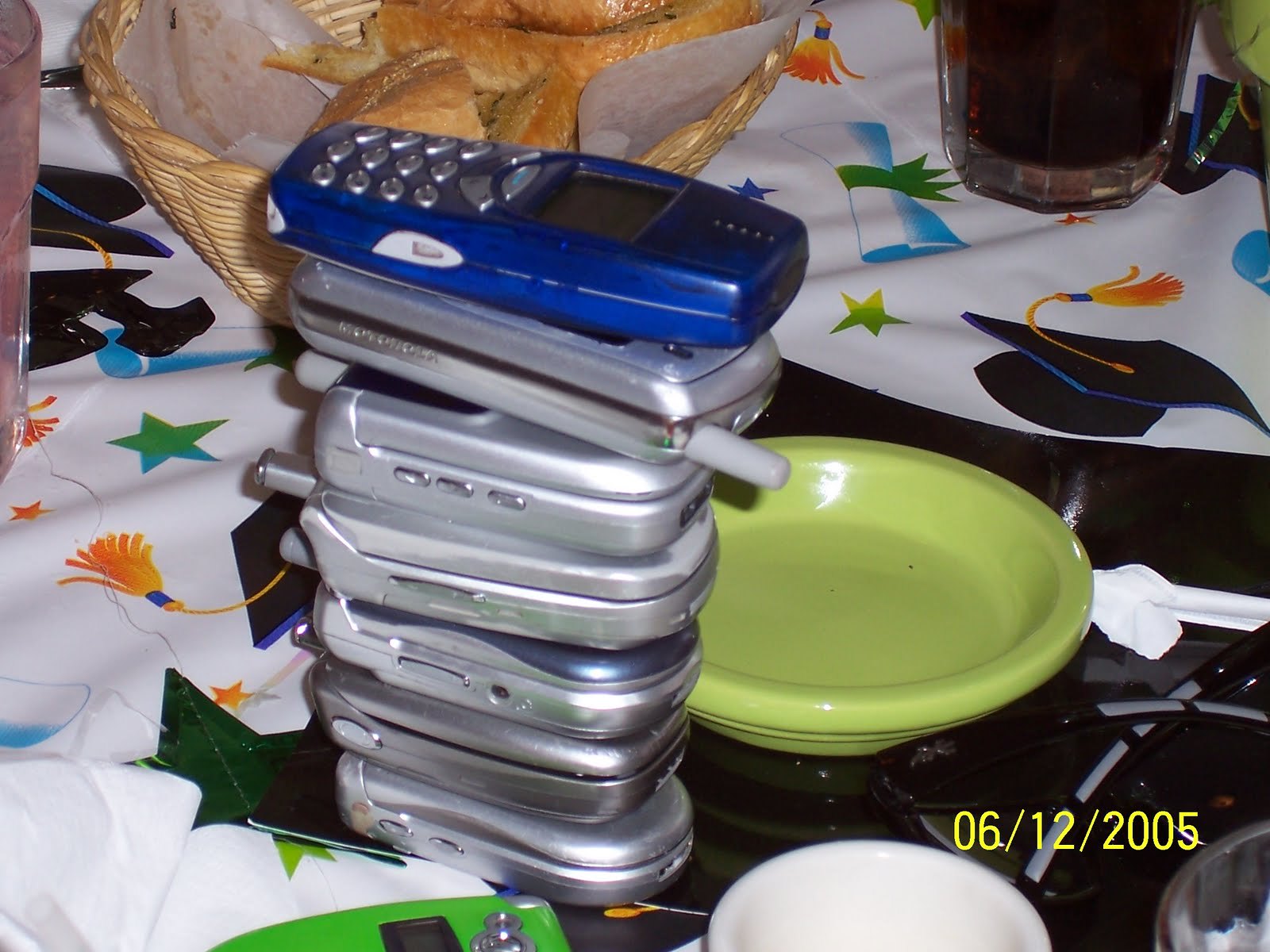The image captures a nostalgic scene of seven antiquated cell phones arranged on a table adorned with a graduation-themed tablecloth, featuring decorative caps, diplomas, and stars. Six of the phones are silver flip phones, meticulously stacked in a tower, while the seventh, a blue non-flip phone with silver buttons and a black screen, crowns the pile. To the right of the phones lies a small light green saucer and a nearby yellow dish. The table also hosts a glass with a dark beverage on the upper right, a white mug, and a wicker basket filled with rolls in the upper left. A straw wrapper is casually placed near the basket. At the bottom right of the image, the date "06-12-2005" is visible, marking the moment frozen in time.